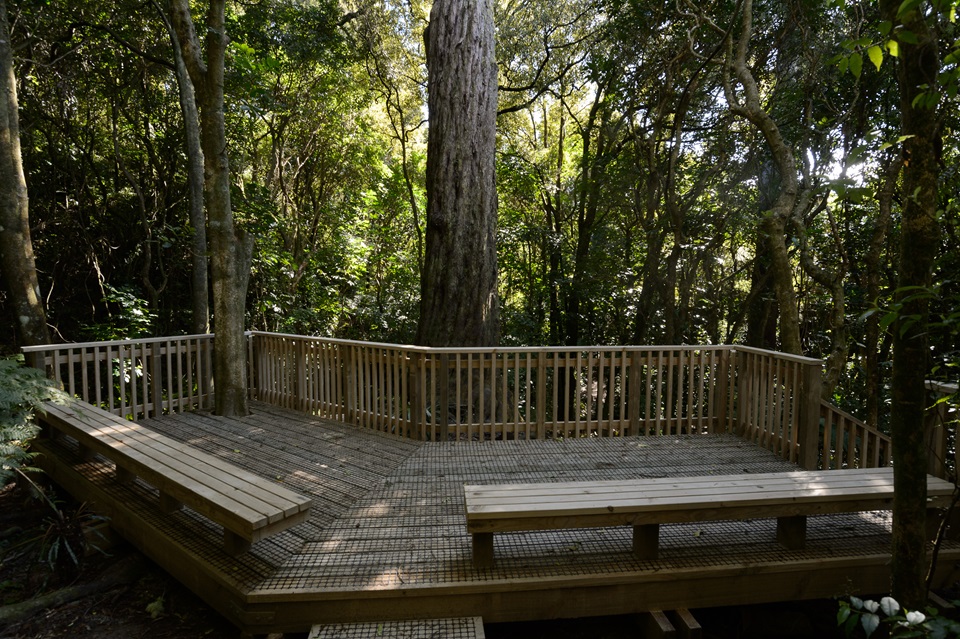This is a detailed color photograph of a large wooden deck situated in a densely wooded forest setting. The expansive deck is constructed entirely from wood and features a railing along most of its sides. There are wooden stairs leading up to the deck on the right side of the image. The deck includes two long wooden benches located closest to the camera, offering seating options for visitors. Notably, the structure is built around a prominent tree, with the tree's trunk emerging through the base at the far left corner of the deck, seamlessly integrating nature into the design. In the background, a multitude of trees create a canopy that allows only sparse sunlight to filter through, emphasizing the secluded, forested atmosphere.